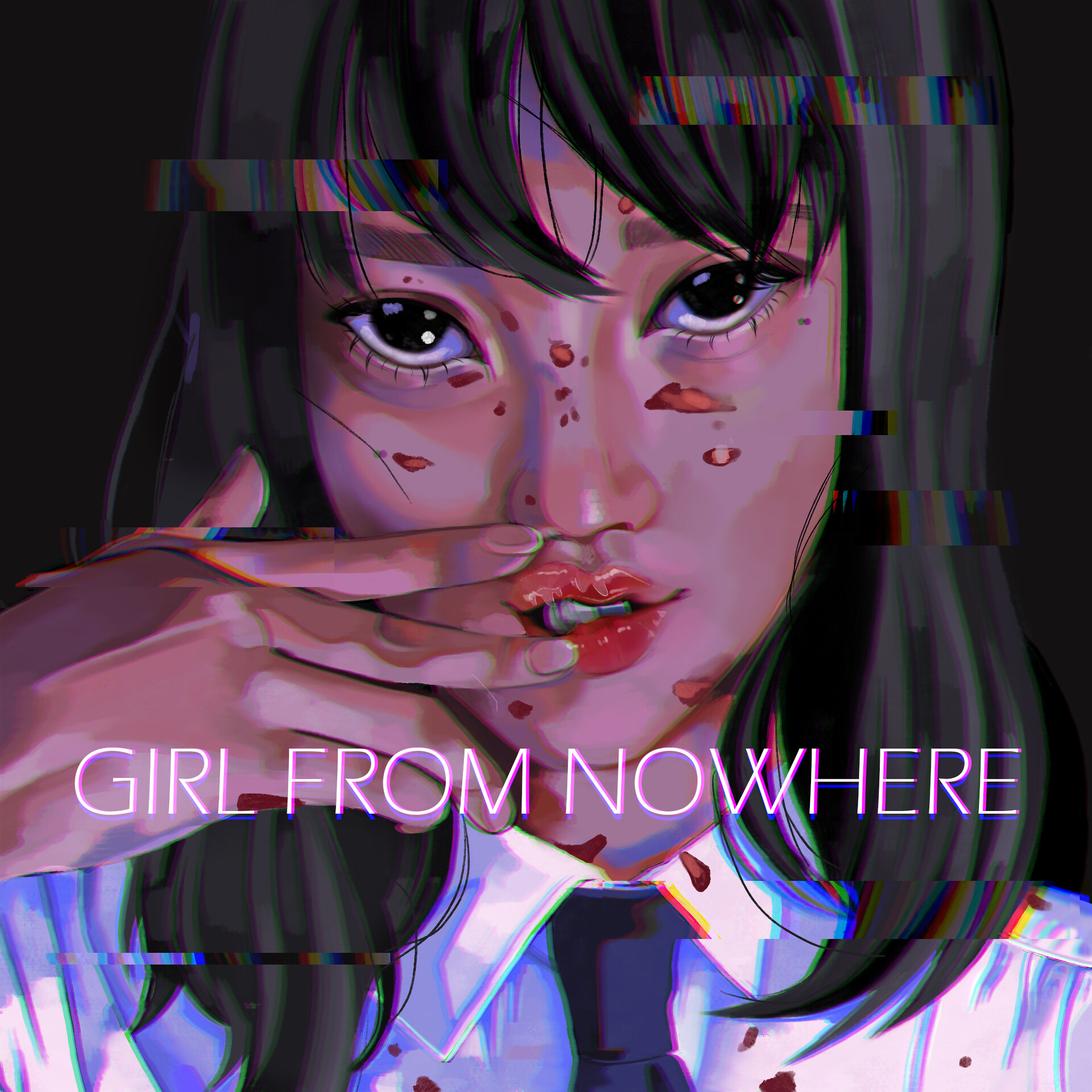This digitalized anime-style image features a close-up of a young Asian woman's face and upper shoulders. She has long black hair with bangs that fall across her forehead and large, dark eyes. She wears a collared white button-up shirt with a black tie, which is fully buttoned to the top. Her hands are raised to her face, with one finger on either side of her lips, slightly pulling them apart. Her lips appear to be red or slightly orange, and she is splattered with a red substance, likely meant to represent blood, across her face and upper body. The image also features thin, white text in all caps just below her chin, reading "GIRL FROM NOWHERE" in a sans-serif font.